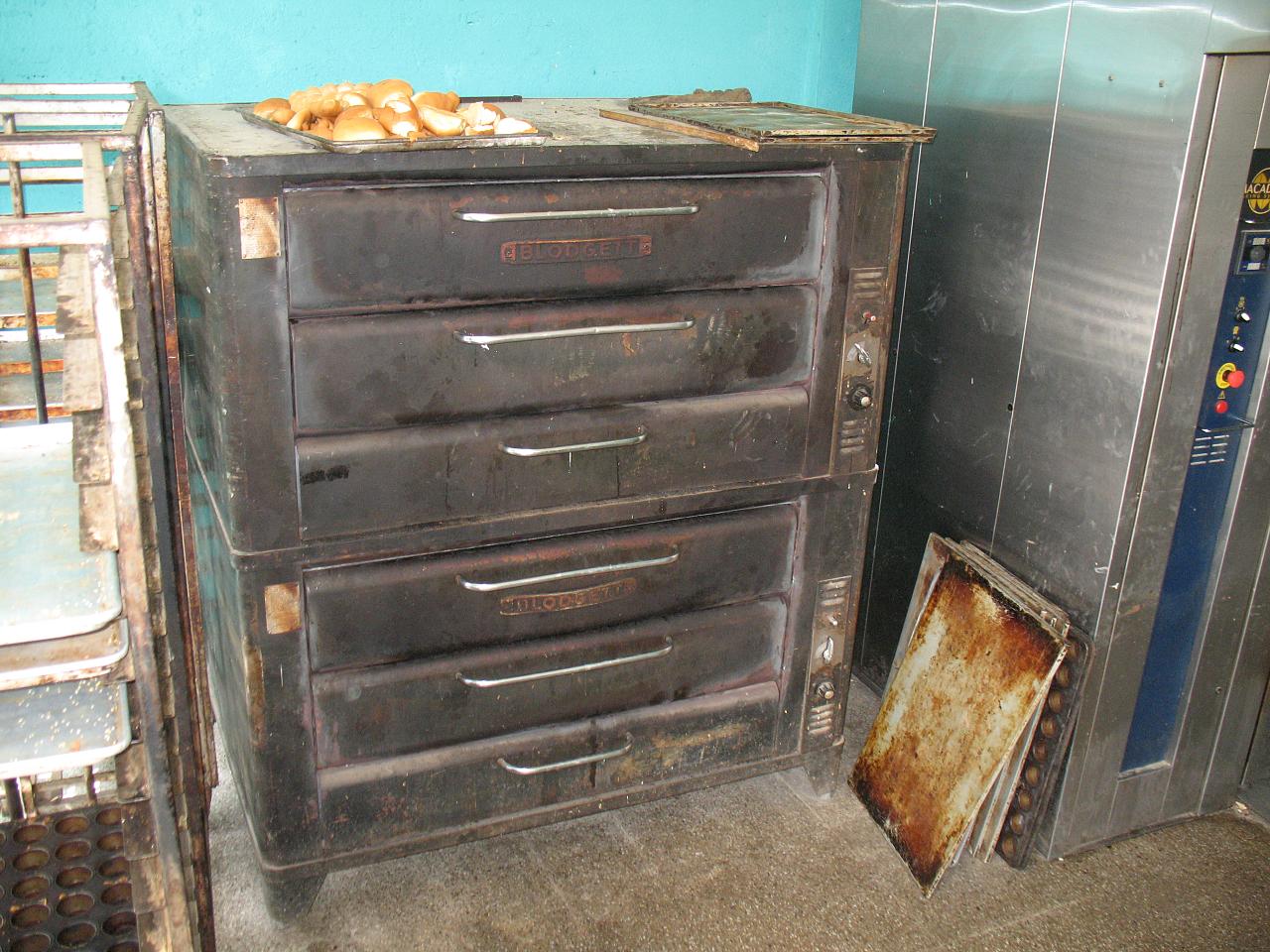The image depicts the interior of a grimy, industrial kitchen, likely a bakery given the presence of various baking equipment. Centrally featured is a large, metal industrial oven with six pull-out drawers resembling a dresser, designed for baking multiple layers of goods simultaneously. Atop this oven, a cookie sheet holds an assortment of bread and buns. To the oven's right stands a large silver appliance, potentially a fridge or another piece of industrial kitchen equipment, covered in knobs and buttons for various settings. On the left side are several racks likely used for cooling freshly baked items. The kitchen's cleanliness is questionable; the floor is dirty and brown, and multiple trays stacked against the equipment appear scorched and never properly cleaned. Additionally, the oven itself shows considerable wear and tear, contributing to the overall unkempt and aged appearance of the space. The back wall of the kitchen contrasts with its bright blue color, adding a stark backdrop to the otherwise grimy scene.